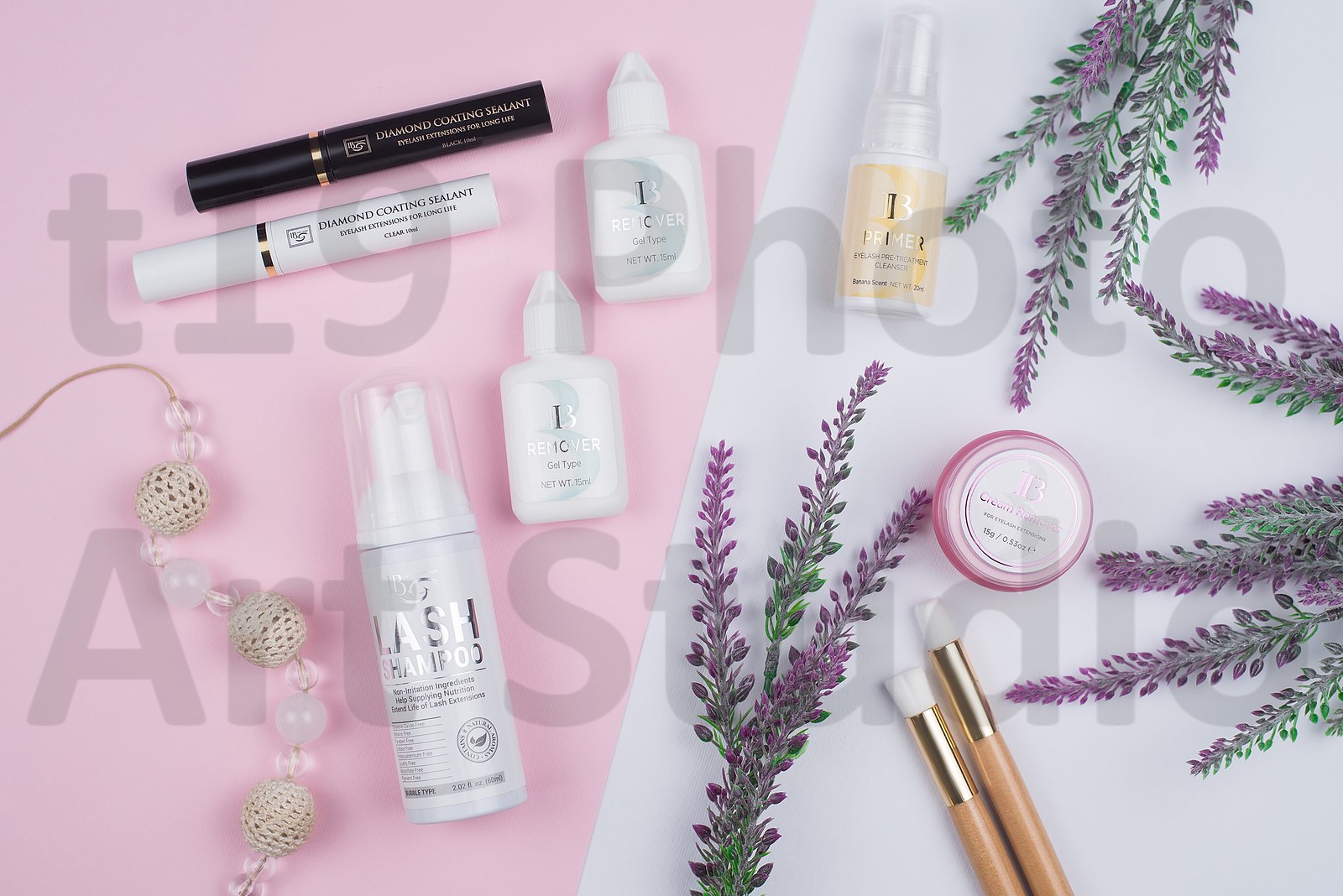A professionally composed photograph captures an elegant array of beauty products arranged against a two-toned background with a diagonal division. The left side is a soft pink, while the right side is a light gray.

On the pink side:
- There are two mascara tubes, artistically angled. The tube at the top is black, leaning gently to the left. Below it, a white tube matches the first in design, both featuring a gold band near their lids.
- Adjacent to the mascaras are two identical white eyedropper bottles, each marked with a prominent number "1".
- Below these, a mini shaving cream pump container is showcased, complete with a transparent lid revealing a white pump beneath. The container has "Lash" written on it, indicating its use for eyelashes.
- A delicate necklace lies nearby, adorned with a mix of beads. Three crocheted beads share space with translucent and transparent beads, possibly made of white jade or opaque and clear glass.

On the gray side:
- A short skin care product bottle is visible, topped with a transparent spritz-style pump lid. It bears a pale orange label with gold lettering.
- In the center sits a small, round jar, appearing to hold a reddish substance. It has a screw top and likely contains less than an ounce.
- Two makeup brushes lie diagonally beside each other, their light wood handles and gold-colored ferrules gripping short, white bristles.
- Lavender sprigs, possibly artificial, add a touch of grace, extending from the top right and various positions within the photo.

A large watermark reading "t19 Photo Art Studio" spans the image, adding a watermark.